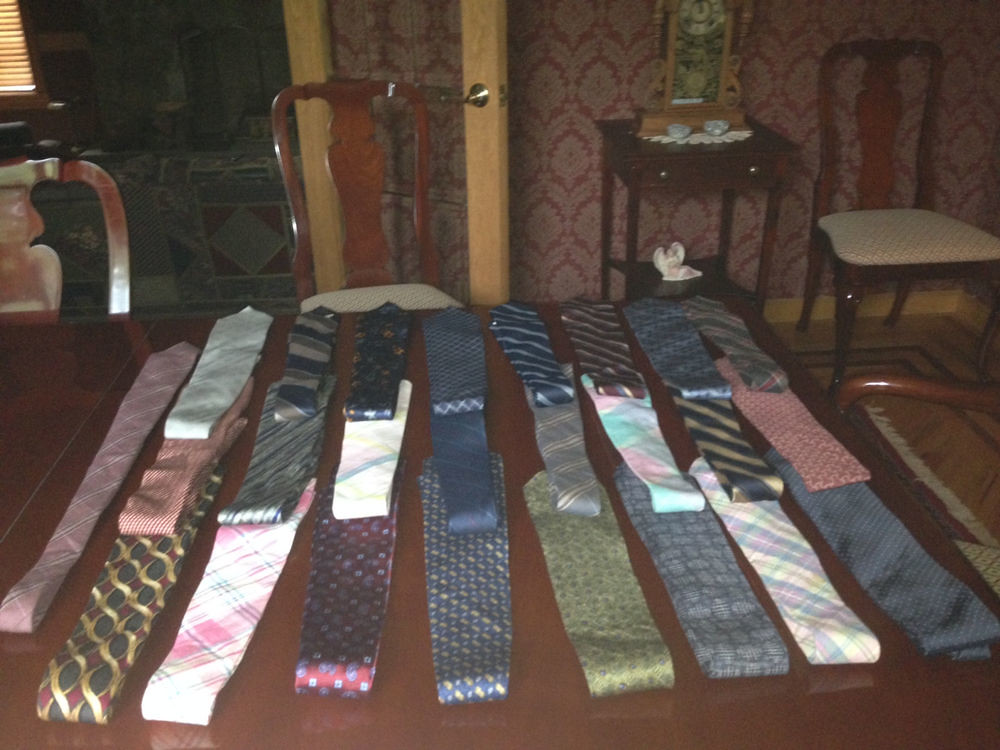The image depicts an antiquated dining room within a very old house, characterized by its outdated decor. The focal point is a dark cherry wood dining table surrounded by matching dark cherry wood chairs with white fabric cushions. Spread across the table are neatly arranged neckties—approximately twenty-five in total—with their pointed ends facing the back wall. The ties showcase a variety of colors and patterns, including stripes, dots, pastels, and muted tones, predominantly made of silk. The wallpaper is notably busy and geometric, with a dark red and white filigree or diamond pattern, encompassing the upper right quadrant and extending across the top center. To the top left, a door opens to another room where an old-fashioned couch with outdated print is visible. Additionally, other furnishings in the room include a small dark wooden table with a doily and possibly a tall clock, and another chair of the same design as those around the table. The overall atmosphere conveys a sense of nostalgic charm and historical richness, enhanced by the interplay of light possibly streaming in from a subtly hinted window.